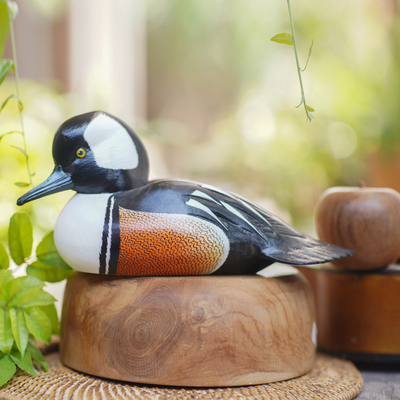A meticulously painted duck figurine, crafted from stone or a similar material, sits gracefully atop a smooth, wooden, upside-down bowl. The duck features striking black wings adorned with white highlights, while its side wing is detailed with a rusty hue and a white edge. Its chest is painted white, and a white patch graces the side of its head, contrasting with the overall black of its body and beak. The duck's eye glimmers in golden color, complete with a detailed central dot. Beneath the wooden bowl rests a round, basket-brown placement pad. Adjacent to this setup, on the right, lies another brown bowl containing a small, polished wooden apple. The background, albeit blurry, reveals a window with verdant greenery and a few branches framing the scene, emphasizing the focus on the duck and its elegant perch.